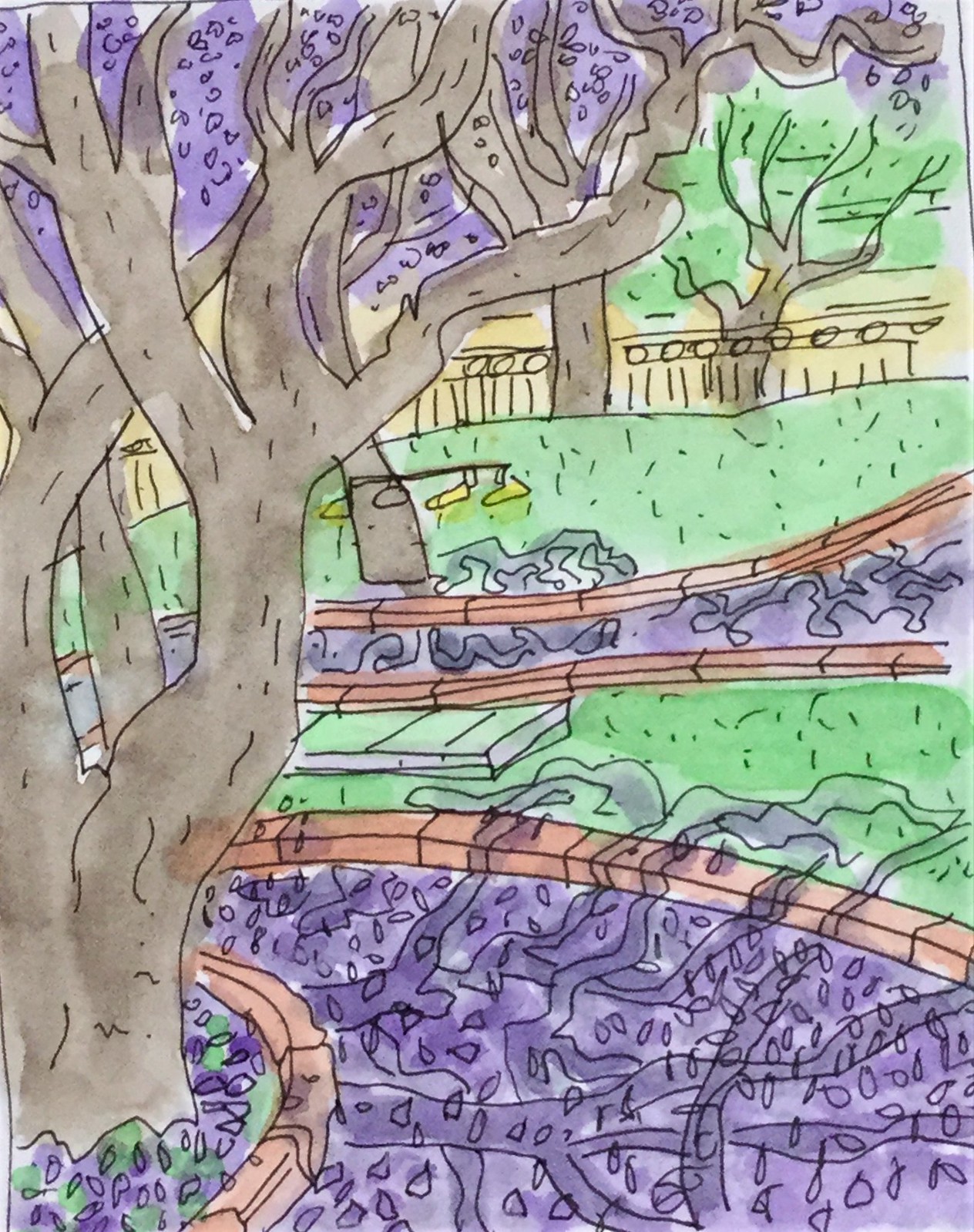This image is a high-quality scanned picture of a watercolor painting depicting a vibrant park scene. Dominating the left side, a large tree with purple blossoms extends its branches over the area. In the background, another tree features green foliage. A detailed grass path winds through the scene, bordered by areas delineated with bricks, where the ground-level purple flowers mirror the blossoms above. Tree roots create intricate shadow patterns along the path. 

A contrasting gray tree stands on the right, encircled by a hedge of bricks and bordered by a lightly green walkway. Patches of grass weave through the settings, interspersed with quaint brick ridges. The painting skillfully integrates an array of elements: outlined black ink defines various features, including light blue ponds outlined sharply, and a stone path shaded in gray. A fence, composed of quick, sketchy lines and circles, frames the scene in the distance, while black ink and watercolor render a central structure in yellow. Trees at various depths showcase trunks of brown and gray, with leaves in the light blue hue, harmonizing the natural setting.